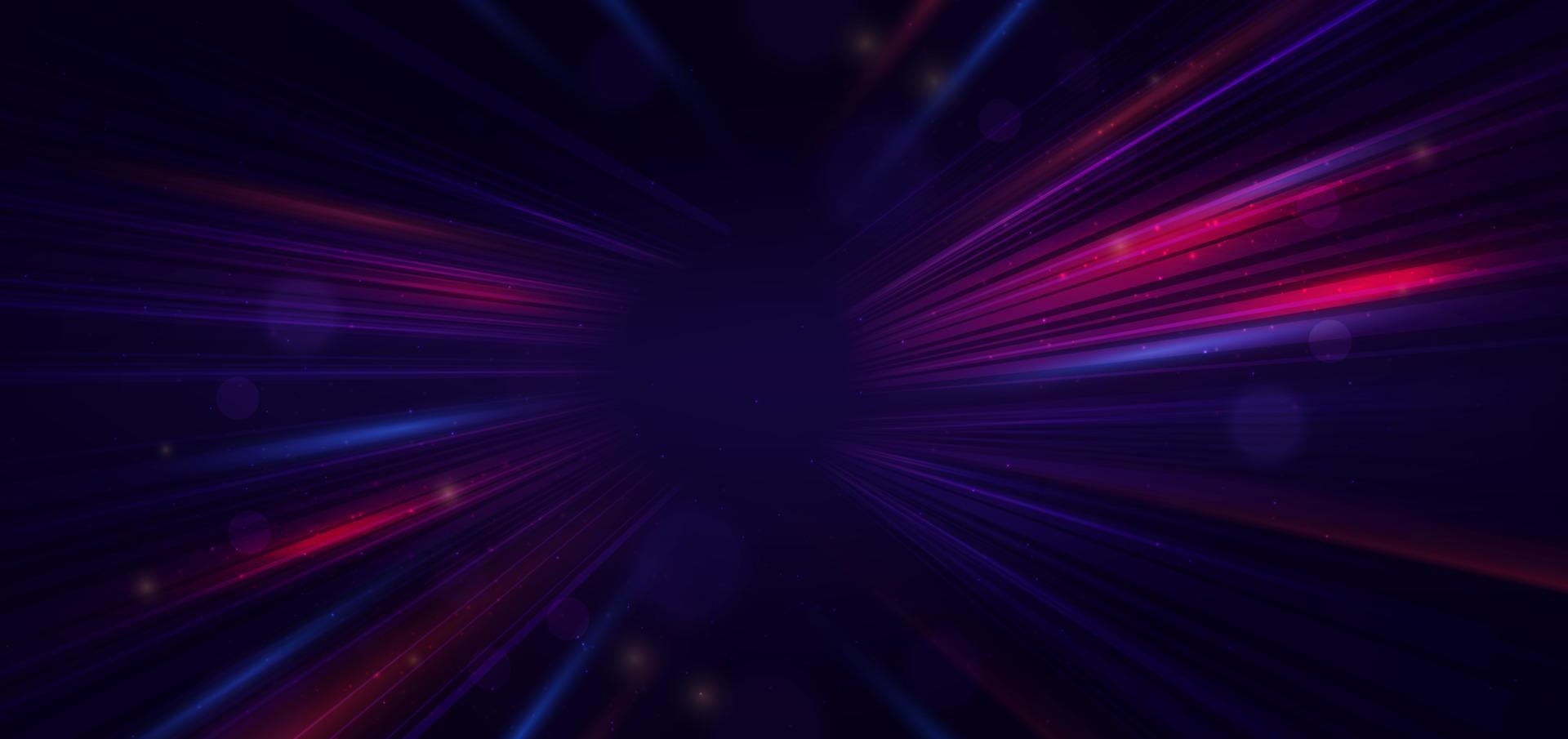The image is a rectangular graphic design set against a predominantly dark or black background. At its center, there is a vibrant circular nexus from which rays of colorful light radiate outward in all directions, spanning from the middle to the edges of the photo. These rays are a striking array of colors, including shades of purple, pink, magenta, blue, and sometimes muted purplish-pink, creating an eclectic, random pattern with no fixed order. The rays vary slightly in size but generally maintain similar widths, contributing to a dynamic yet cohesive visual effect. Scattered among the rays are specks and small orb-like splotches in shades of blue, purple, pink, and even orange, adding depth and complexity to the design. The photo is devoid of any text, people, or other distinguishable objects, focusing solely on the vivid interplay of light and color against the dark background.